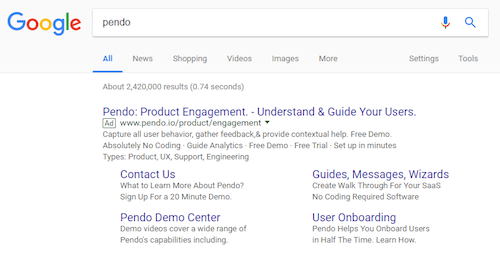The screenshot showcases a Google search page with the following elements:

- The upper left-hand corner features the iconic Google logo with its blue, red, orange, and green letters.
- Below the logo is the search bar with the query “Pendo” entered (spelled as P-E-N-D-O).
- The navigation bar beneath the search bar includes options: "All" (which is underlined), "News," "Shopping," "Videos," "Images," "More," "Settings," and "Tools."
- The search results indicate approximately 24,420,000 results found in 0.74 seconds.
- The first result is a sponsored advertisement for Pendo.io. The ad headline reads: "Pendo: Product Engagement, Understanding Your Guides and Users."
- The ad description elaborates on Pendo’s capabilities, such as capturing all user behavior, gathering feedback, and providing contextual help. It highlights features like a free demo with no coding required, various guides, analytics, free trial availability, and the ease of setup in minutes. Pendo supports multiple types, including product, UX, support, and engineering.
- Additional details include a call to action to contact Pendo for more information, sign up for a 20-minute demo, and explore various features like guides, messages, wizards, and software walkthroughs without coding.
- The Pendo Demo Center is mentioned, offering demo videos that cover a wide range of Pendo's capabilities, including user onboarding, emphasizing that Pendo helps onboard users in half the time.